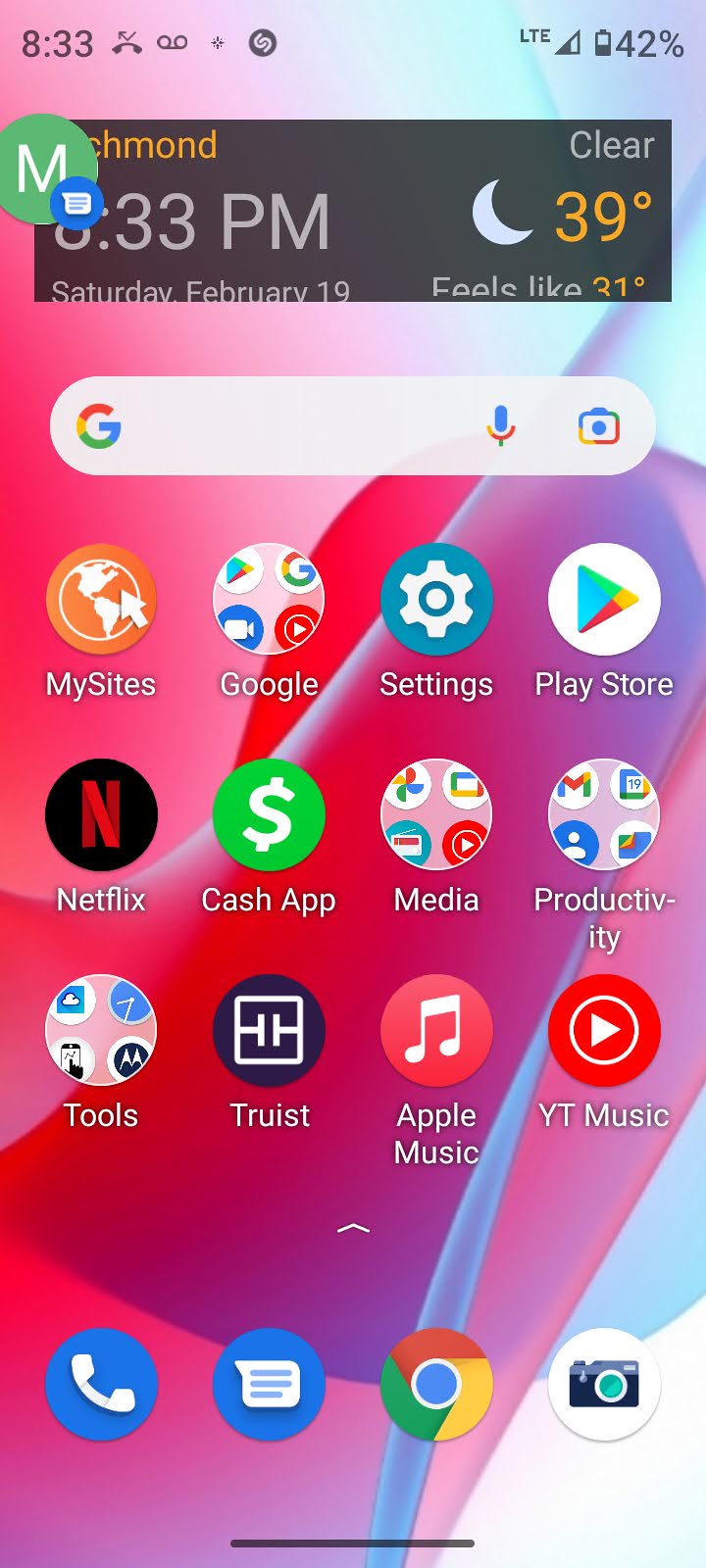This image is a screenshot taken from an Android phone, showcasing the home screen layout. At the very top left, the time "8:33" is displayed, alongside symbols indicating a missed call and a voicemail notification. The top right shows the battery percentage at 42% and two bars of internet connectivity. Below this, a gray box prominently features the time "8:33 PM" on the left and the temperature "39°F" with a moon icon, suggesting nighttime.

Directly beneath the gray box is an elongated oval-shaped search bar with the Google logo on the left, and icons for voice search and image search on the right. Below the search bar, the screen is organized into three rows of application icons. The first row includes "My Sites," "Google Settings," and "Play Store." The second row lists "Netflix," "Cash App," "Media," and "Productivity." The third and final row contains "Tools," "Truist," "Apple Music," and "YouTube Music."

At the very bottom of the screen, there are four primary application icons. From left to right, they are a phone icon for calling, a message icon for texting, a Google Chrome icon for web browsing, and a camera icon for taking photos. The background of the home screen is a vibrant mix of colors including pink, purple, magenta, white, and light pink, adorned with various abstract shapes.